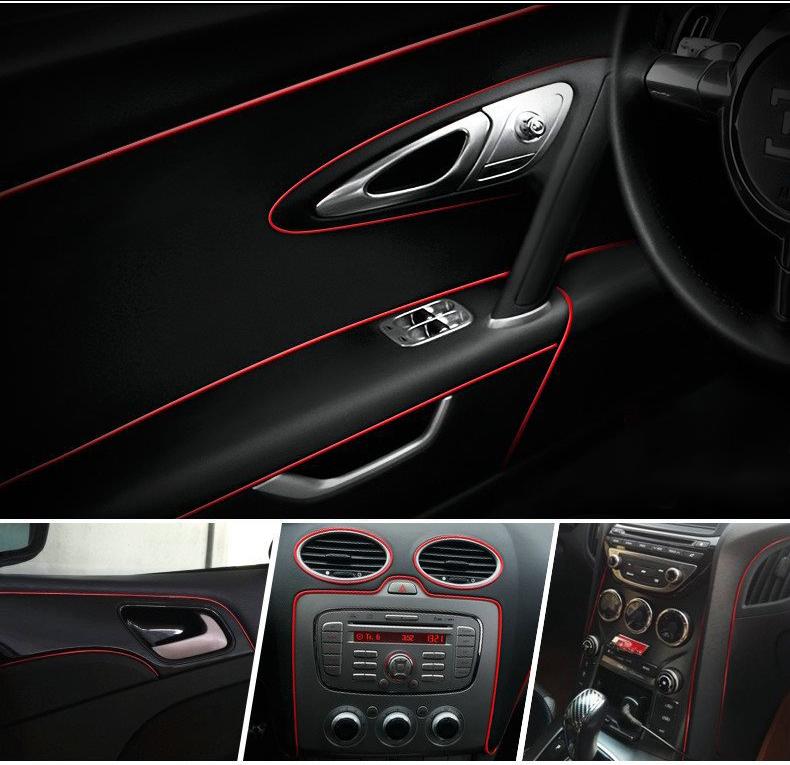The image consists of four photographs capturing the sleek, modern black interior of a vehicle, accented with striking red lines. The largest photo at the top showcases the inside of the driver's side door, complete with a silver door handle, an insignia, and various black buttons set in silver panels. The red accent lines run beneath the window and around the armrest. The edge of the black steering wheel is also visible on the right. Below, the first smaller image on the left appears to be a close-up of a door lock on the passenger side, identifiable by the rearview mirror in the upper left corner. The middle image focuses on the center console featuring the radio, with multiple buttons, a horizontal digital display, and three large knobs, framed by a red outline, and topped with two air vents. The bottom right image seems to show another console, possibly from a different car, or a different part of the vehicle, with additional smaller knobs, vent controls, and the gear shift visible. Each section of the car interior maintains the coherent design palette of black with red detailing, emphasizing its contemporary aesthetic.